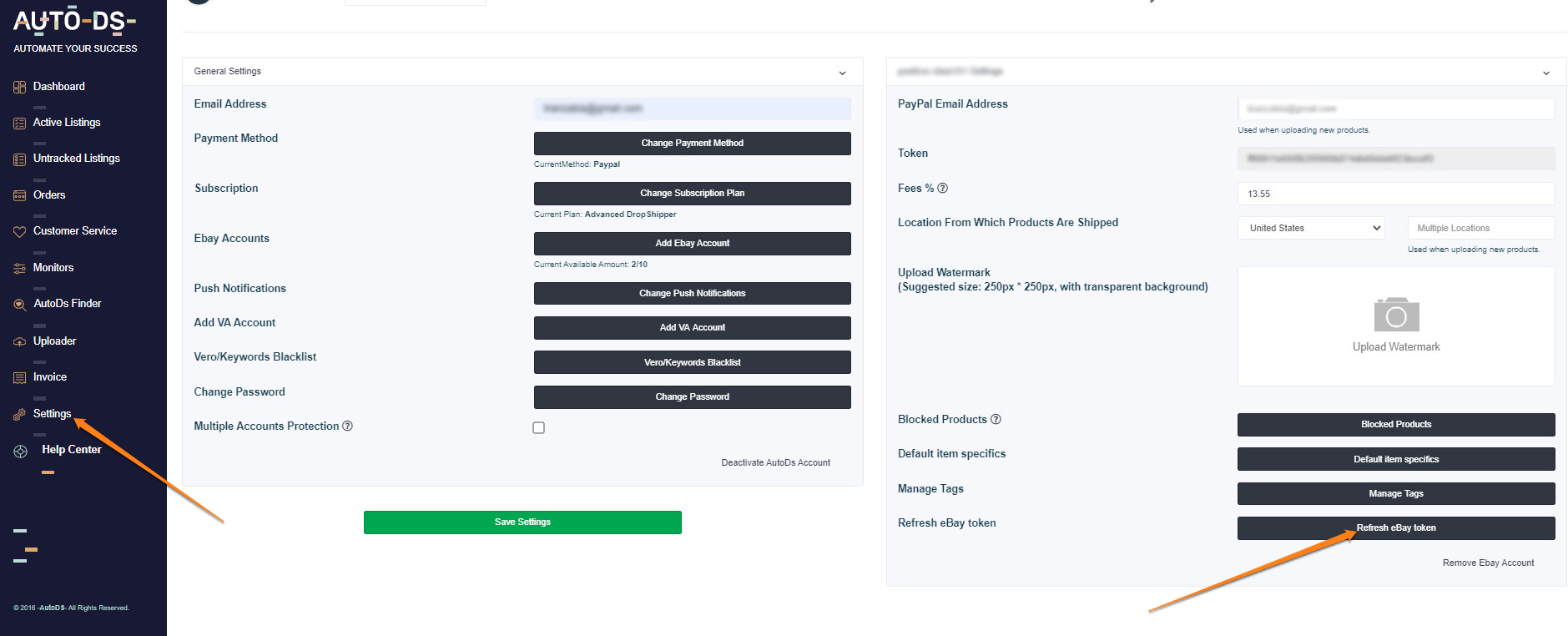The image depicts the user interface of AutoDS, accompanied by the slogan "Automate Your Success" prominently displayed at the top left corner. Below the slogan, there is a vertical menu with a dark, almost black background, featuring white text for each menu item. The menu items listed sequentially are: Dashboard, Active Listings, Untracked Listings, Orders, Customer Service, Monitors, AutoDS Finder, Uploader, Invoice, Settings, and Help Center. An orange arrow points specifically to the Settings option.

To the right of this menu, there are two large informational blocks. These blocks include fields for items such as email addresses and payment methods. In the rightmost block, another arrow directs attention toward a button labeled "Refresh eBay Token," indicating a function to update the eBay connection. The button appears somewhat distanced from the other elements within the block, making it visually isolated.